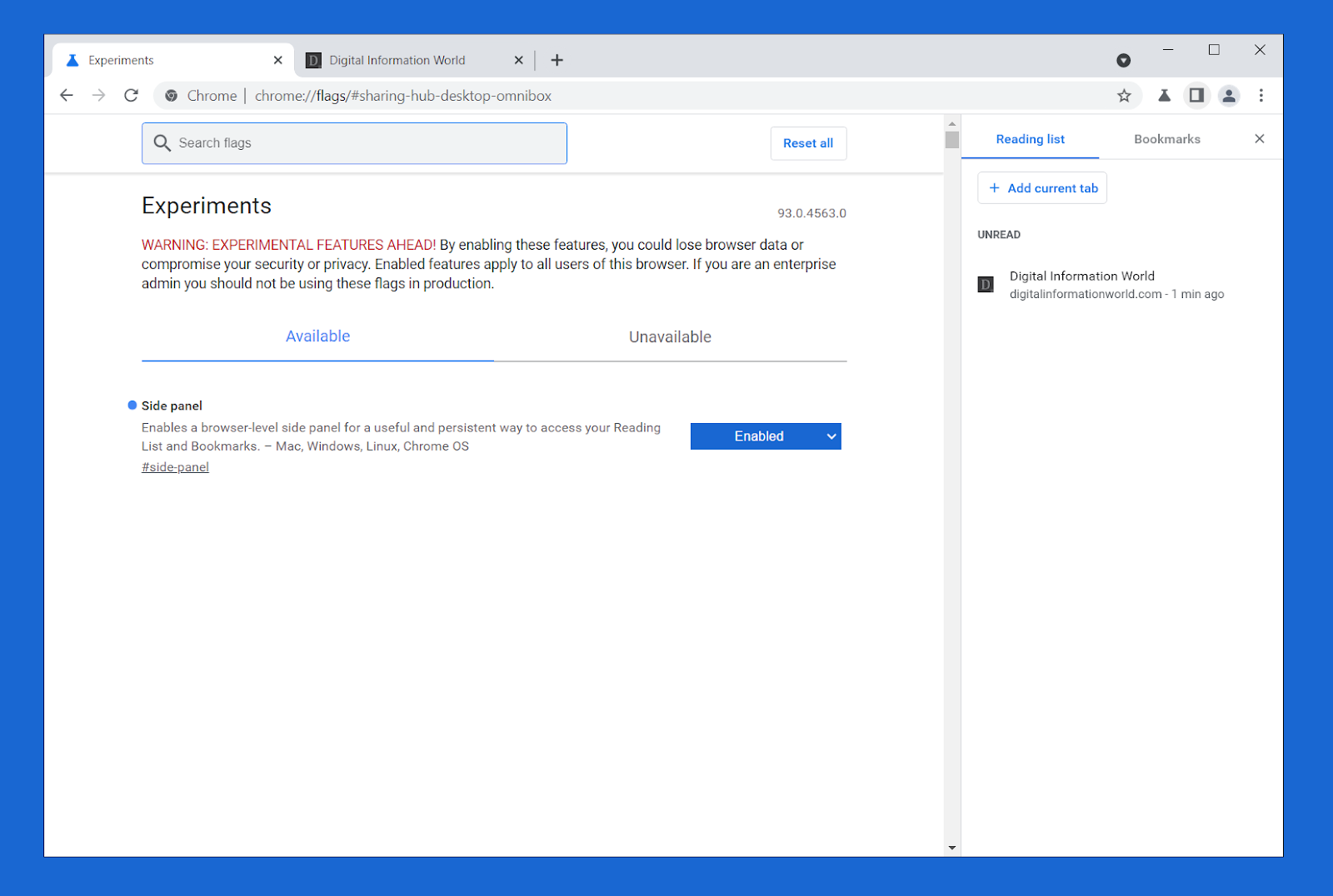The image features a browser window with a predominantly dark blue border. At the top of the window, two Chrome tabs are visible. The first tab, labeled "Experiments," is highlighted in white, indicating it's the active tab. The second tab, labeled "Digital Information World," is gray, signifying it's inactive.

On the right-hand side of the tabs, typical window controls are present: a drop-down arrow, a horizontal line, a square to maximize/restore, and an "X" to close the window.

Directly below the tabs, the browser's navigation bar is displayed against a white background. The back button is black, suggesting it's clickable, while the forward button is gray, indicating it's inactive. The refresh button is also black. The search bar has a gray background with black text. To the right of the search bar, some unidentifiable icons are present.

The main content of the active tab shows a page titled "Experiments." At the top center, a blue rectangular search box with a magnifying glass icon and the text "Search Flags" is present. To the right of this search box, a blue "Reset All" button is situated.

Beneath the search box, black text reads: "Experiments. Warning: experimental features ahead. By enabling these features, you could lose browser data or compromise your security or privacy. Enabled features apply to all users of this browser. If you are an enterprise admin, you should not be using these flags in production."

Following this warning text, further options are listed: "Available," "Unavailable," "Side Panel Stuff," along with additional unreadable information.